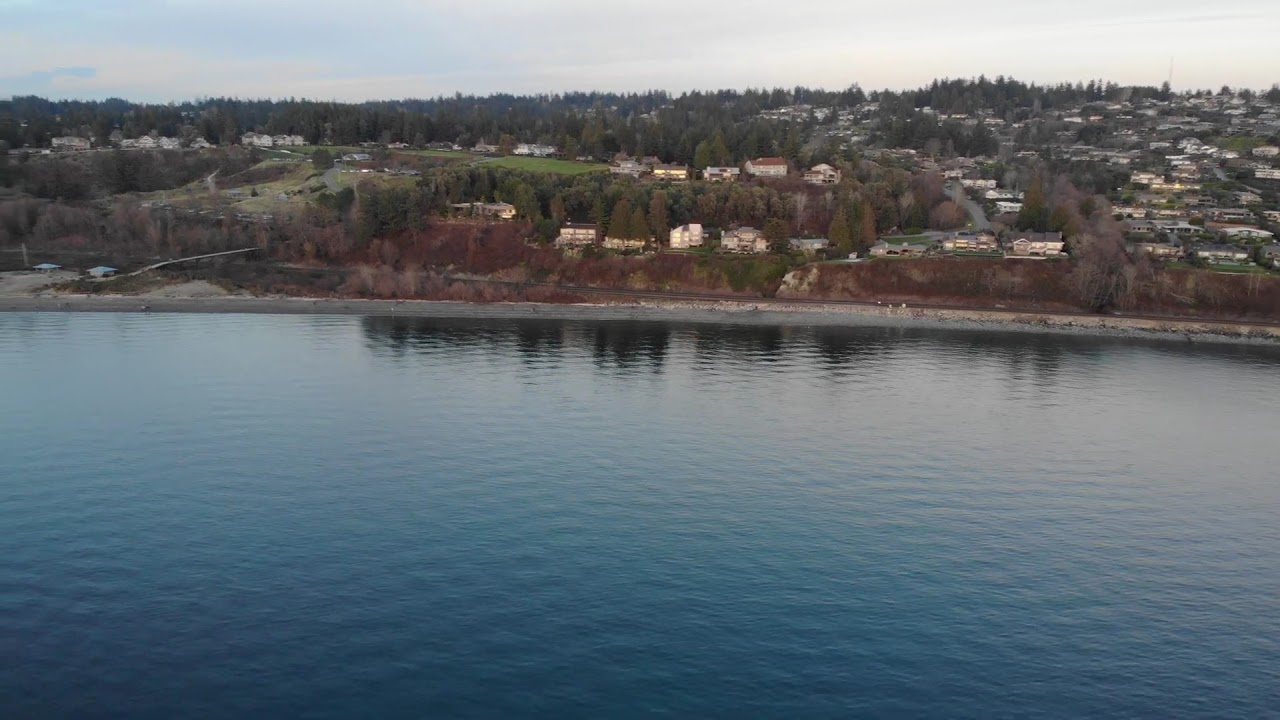Full-color photograph taken outdoors, likely in early fall. This horizontally rectangular image features a large, calm body of water occupying the bottom half, exhibiting gentle ripples without significant waves. Along the shoreline, a white rocky area transitions into a dirt hill, which ascends to reveal rows of large, distant two-story homes nestled among a diverse array of trees. The foliage suggests early fall, with some trees turning shades of red, orange, and yellow, while others remain green or stand bare. The upper half of the image displays a mostly sunny sky with wisps of clouds and reflections of the trees at the water's edge. The setting appears to capture a serene, mid-day scene overlooking what seems to be a large lake, with the natural and built environments harmoniously blending together.